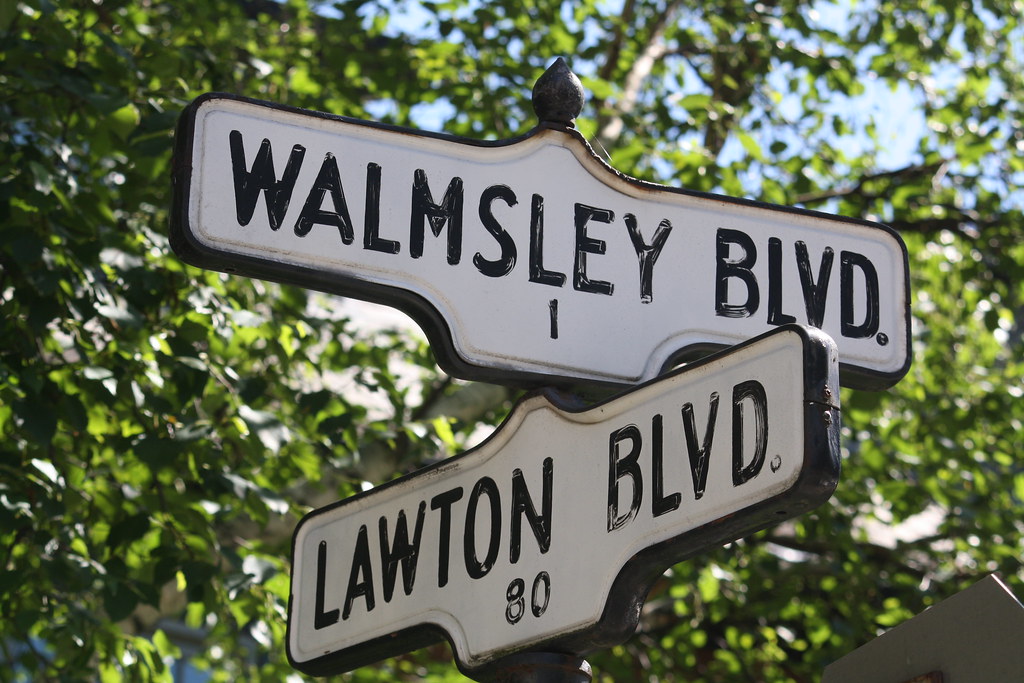The image captures a street corner on a bright, sunny day, characterized by two intersecting street signs. At the top, a white enamel sign with black lettering identifies "Walmsley Boulevard" and displays the number "1" below it. Crossing this, another enamel sign reads "Lawton Boulevard" with the number "80" beneath. Positioned at the junction of these signs is a black, bulbous structure, perhaps a bird, whose authenticity is ambiguous. The background features deciduous trees with visible branches, trunks, and fluttering leaves, set against patches of a clear blue sky. The daylight highlights the scene vividly, with sunlight filtering through the foliage. In the bottom right corner, there’s a triangular white texture, possibly the top of another sign, against a backdrop that includes a beige-colored structure, indicating a house. The street signs are detailed with a black outline accentuating their lettering.